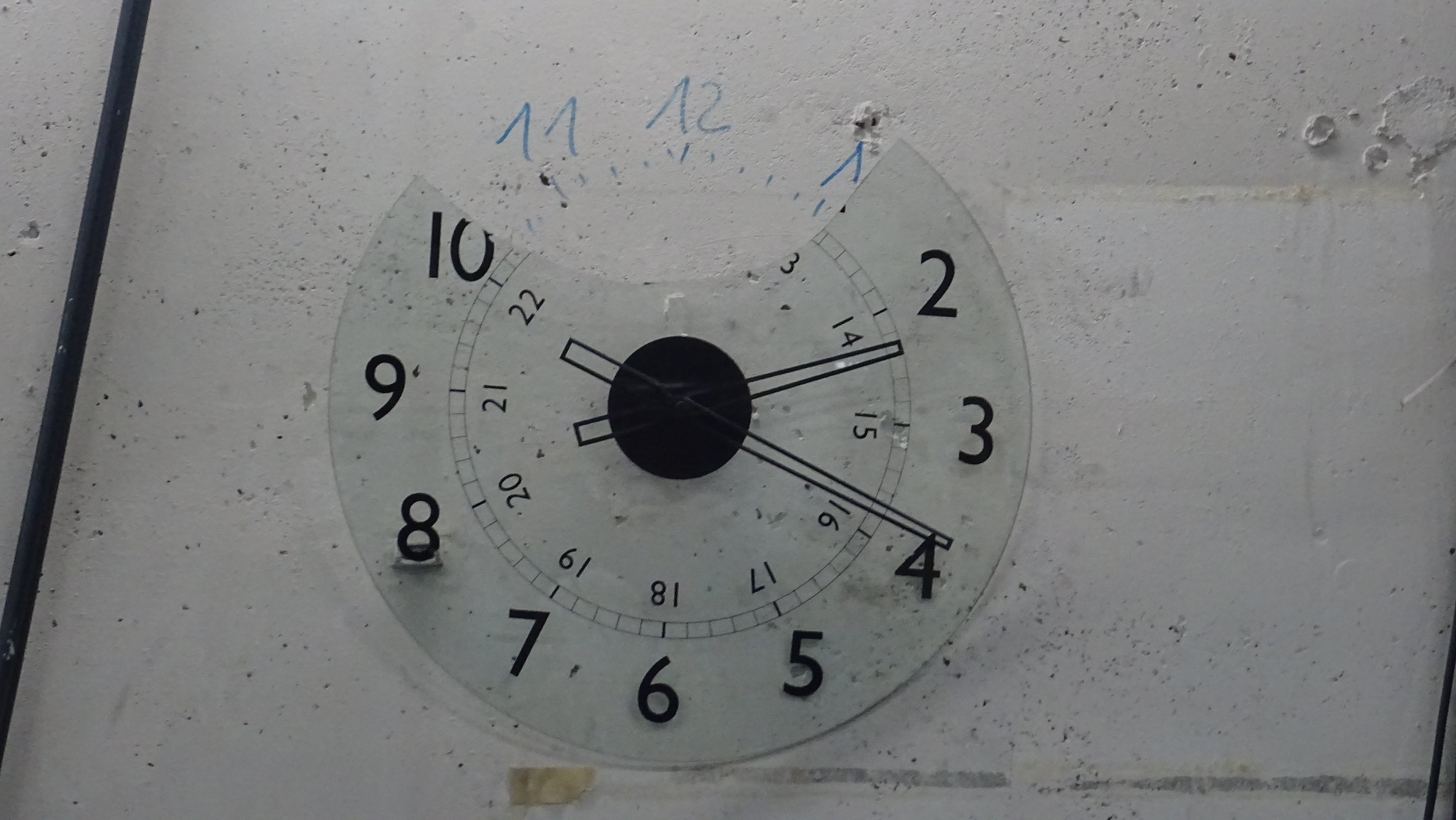This photograph captures a close-up view of an analog wall clock set against a light gray background. The most noteworthy feature of this clock is its unique construction, with numbers, minute, and hour hands all positioned on an entirely clear disc, likely made from plastic or glass. Traditional numerical markers, rather than Roman numerals, encircle the disc. The time displayed on the clock reads approximately 2:19.

An intriguing aspect of this image is found at the top of the clock, where the area that normally showcases the numbers 11 and 12 is broken. Instead of repairing the clock, someone has innovatively written the numbers 11 and 12 directly onto the wall, along with the five-minute increment markers that typically reside between these numbers. This clever adaptation ensures that the clock remains functional despite its damage, creating a visually and conceptually fascinating piece.